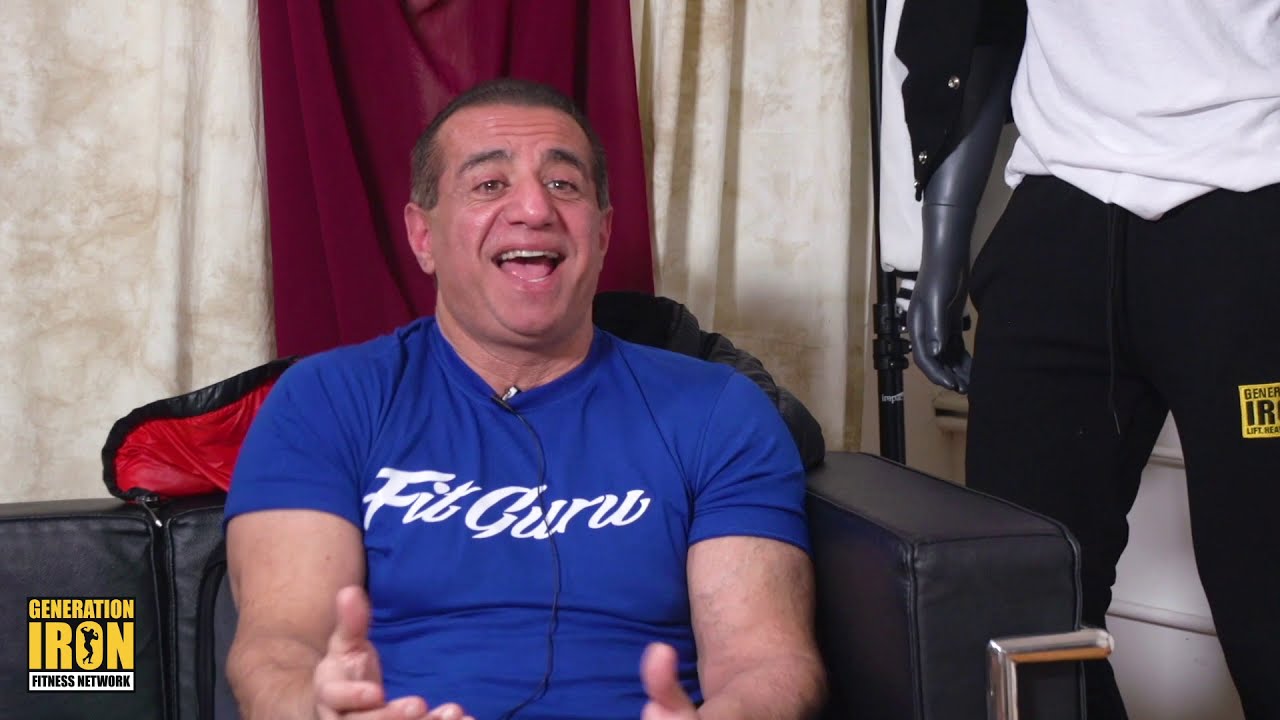The image captures a physically fit, middle-aged man sitting on a dark leather couch with black cushions. He is wearing a blue t-shirt with the text "Fit Guru" in white, cursive lettering. The man appears to be in his mid-50s, with slicked-back gray and brown hair, and he has a clean-shaven face. He is smiling and seemingly in the middle of an interview, indicated by the small black microphone clipped to his t-shirt. 

In the background, a mannequin with gray arms, black pants, and a white t-shirt is partially visible. The setting appears to be indoors, with white curtains featuring brown lines and a dark red curtain. Another item of interest is a red and black jacket situated behind the man. In the bottom left corner of the image, the Generation Iron Fitness Network logo is displayed prominently, with "Generation" in small yellow font, "Iron" in large yellow font, and "Fitness Network" in black font on a white rectangular background. This image likely portrays a scene from a fitness-related interview or discussion.